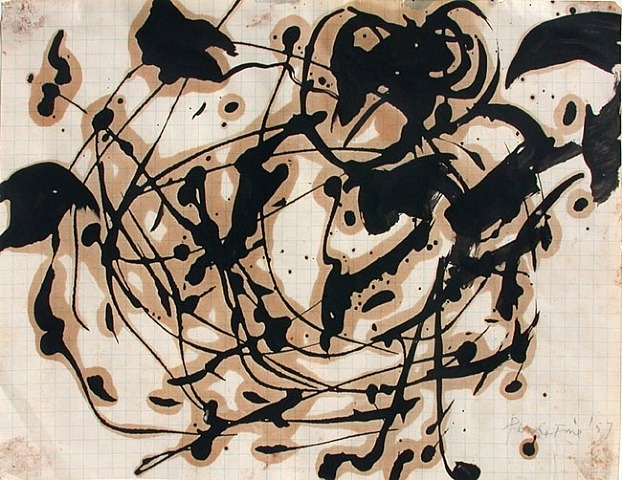The image portrays a modern abstract painting on a gridded white background, which features faint blue or possibly gray lines forming small squares. The centerpiece of this artwork consists of splashes and swirls of dark black paint, applied in a haphazard, expressive manner with many interconnected lines and dots. These black elements are most heavily concentrated in the top half of the painting. The underlying areas behind the black splashes have a brownish or coffee-stained appearance, suggesting the paint bled into the surface, which might be slightly off-white or aged paper. Additionally, there's faint, unreadable text near the bottom, with only the letters "P," "G," and "F" discernible. The painting does not aim to represent any realistic image but rather invites viewers to appreciate the randomness and aesthetics of its application.